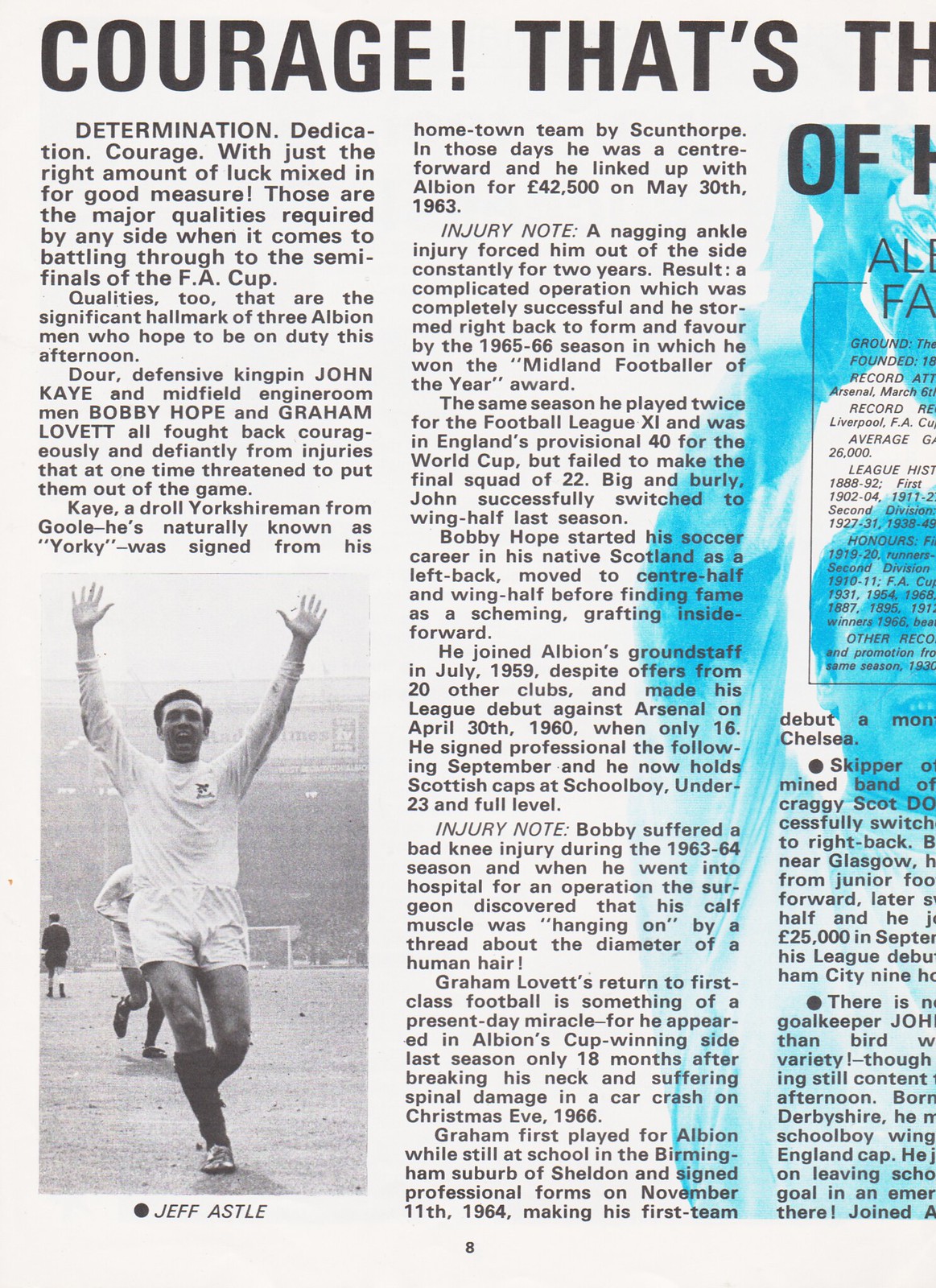The image is a rectangular photograph or cutout of a newspaper article, predominantly in black and white, with a significant smear of blue ink or paint on the right-hand side towards the top. This smear slightly obscures the article. At the bottom left of the image, there is a small black-and-white photograph of a soccer player identified as Jeff Astle, with his hands raised in celebration, possibly suggesting a victory or a goal. The main article text begins with bold black lettering stating "courage!" followed by partial words "that's TH," making the complete headline unclear. The visible part of the article starts with an inspirational message: "determination, dedication, courage...with just the right amount of luck mixed in for good measure" and goes on to discuss the qualities needed to progress in the FA Cup, listing specific players like Doar, John Kay, Bobby Hope, and Graham Lovett. The page's aesthetic suggests it is from an old sports magazine or newspaper, emphasizing its historical context through its monochromatic scheme and detailed narrative on football.